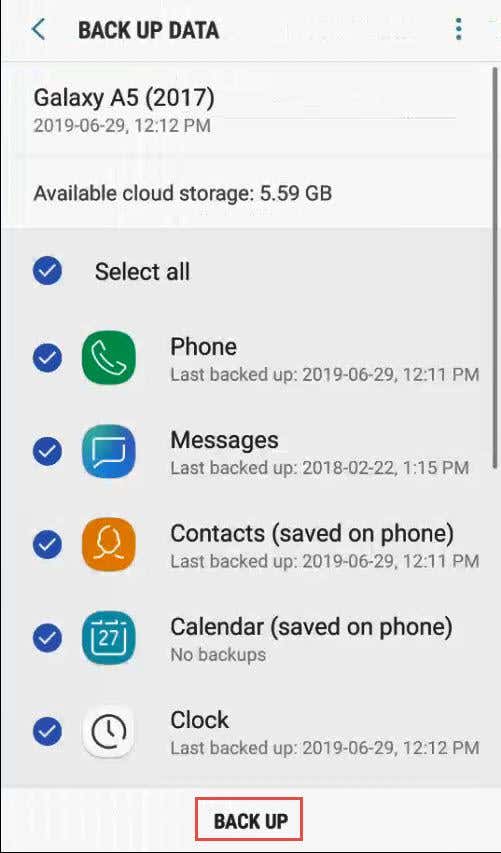The image depicts a screenshot of a cell phone screen, specifically showing a data backup interface. The background at the upper portion is light gray, transitioning to a darker gray in the middle and bottom sections, and finally to white at the very bottom.

At the top left, black text reads "Backup Data." Just beneath this, the phone model "Galaxy A5 (2017)" is displayed, followed by the date "2019-06-29" and the time "12:12 p.m." Further down, the available cloud storage is indicated as "5.59 GB."

The interface features six blue circles, each with a check mark symbol, representing different backup options. These options, listed from top to bottom, are "Select All," "Phone," "Messages," "Contacts," "Calendar," and "Clock." Each of these categories (except for "Calendar") includes the date and time of the last backup, while the "Calendar" option states "No backups."

On the right side of the screen is a gray scroll bar for navigating through the options. At the bottom of the screen, enclosed in a red rectangular border, is a button labeled "Backup" in black text. The entire image is framed with a thin black line along the bottom and left-hand side, defining the edge of the screen.